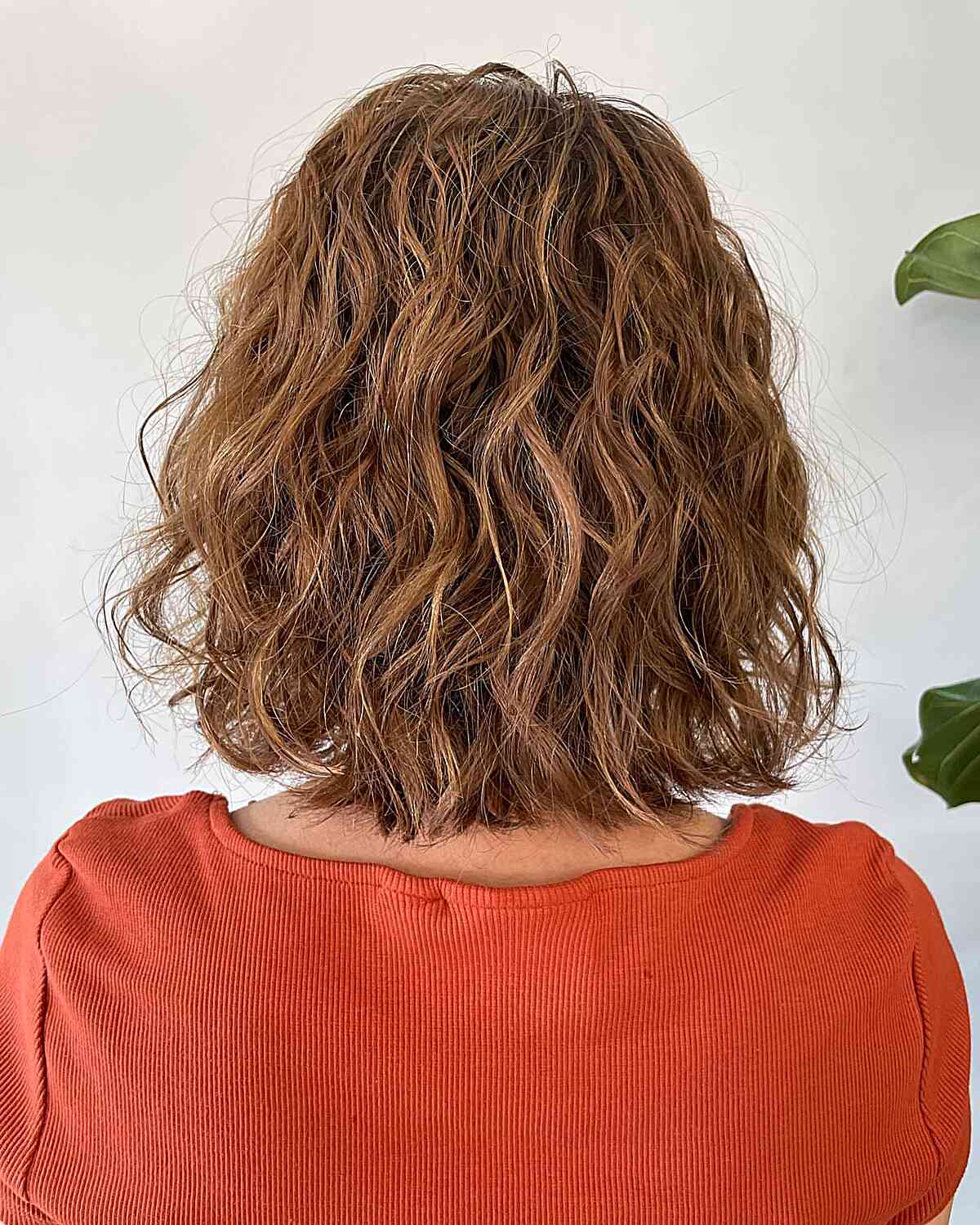The photo depicts a woman sitting with her back to the camera, facing a white wall. Her hair is light brown with a hint of reddish or blondish tones, styled in shaggy waves that rest just above her shoulders. It appears to have some product in it, giving it a scrunched, textured look. She is dressed in an orange top with a wide neck, exposing part of her shoulder and some of her upper neck. The fabric of the top has tiny, vertical woven stripes, reminiscent of a corduroy-like texture. To the right of her, large leaves from a plant extend into the frame, with one leaf situated just above her shoulder and another near the top of her head. The overall composition of the image is slightly taller than it is wide.